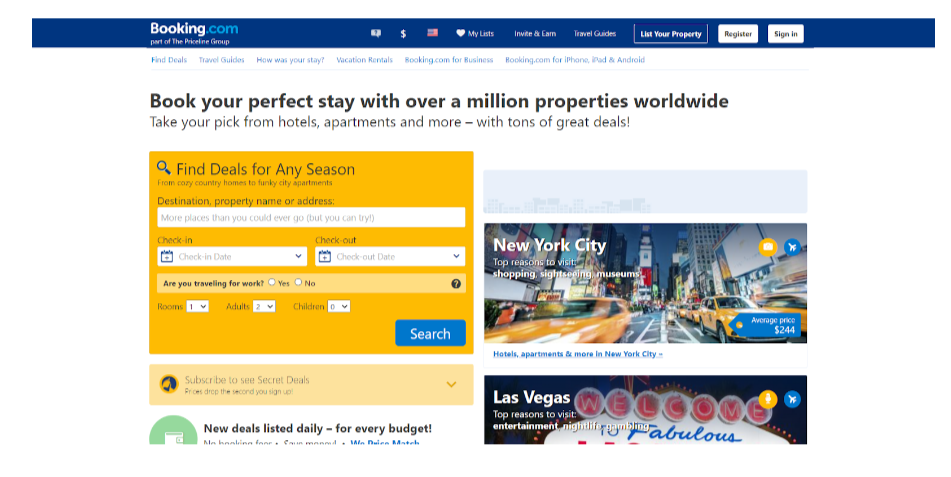The screenshot captures the Booking.com website interface. At the top, there is a prominent blue horizontal bar. On the left side of this bar, the text "Booking.com" is displayed in bold white font, set against a blue backdrop. Adjacent to this area are small icons and text that appear to be too tiny to discern clearly, amidst a section with white and light blue writing.

Centered a couple of lines below, the slogan "Book your perfect stay with over a million properties worldwide" is prominently displayed in black text. Beneath this, a gray description states, "Take your pick from hotels, apartments, and more—with tons of great deals!"

Further down, the layout is divided into two sections. The left section features a yellow background, with a gray magnifying glass icon in the upper left corner accompanied by the text "Find deals for any season." Below this, there is a horizontal white search bar followed by two white rectangles designated for entering start and end dates.

The right section displays a series of rectangular images. At the top, a light blue rectangle contains the text "New York City" in white, situated in the upper left corner of a photograph depicting a city street and buildings. Below this is another photo, of the famous "Welcome to Las Vegas" sign, with the text "Las Vegas" indicated in the upper left corner.